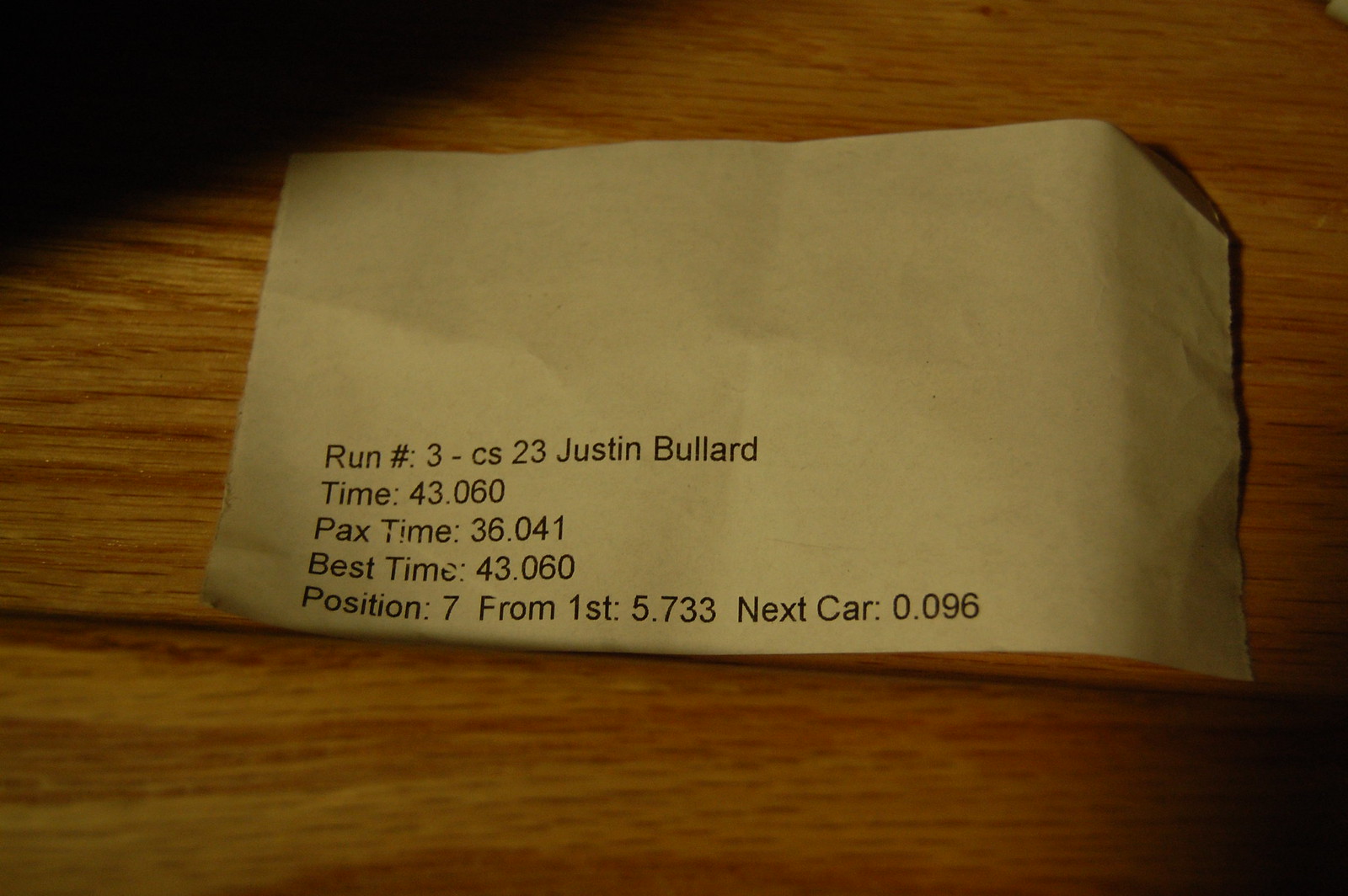The photograph captures a rectangular piece of brown cardstock-like paper resting on a wooden table with pronounced shadows creating a dramatic effect. The table, with a visible wood grain, frames most of the image except for the top left and bottom right corners, where shadows slightly obscure the view. The paper itself features predominantly in the lower-left half, typographically printed in black text. It details the results of an auto race, stating: "Run number: 3-CS23, Justin Bullard." Below this, specific times and positions are listed: "Time: 43.060," "PAX time: 36.041," "Best time: 43.060," "Position: 7 from first, 5.733," and "Next car: 0.096," detailing the performance metrics of the driver, Justin Bullard.